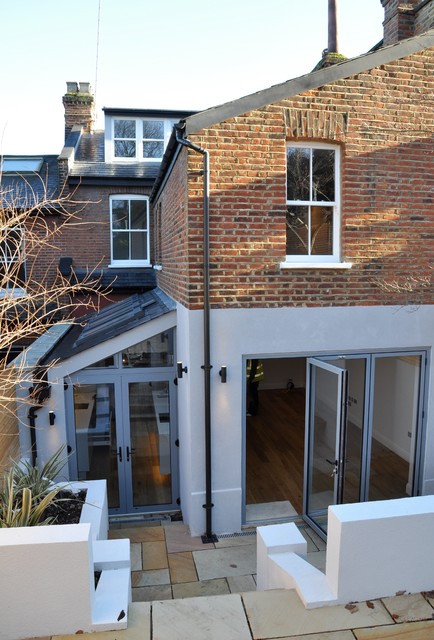The image showcases the back angle of a beautiful two-story brick house in an urban setting, taken during a clear mid-morning. The upper portion of the house is built with brown bricks, featuring two visible windows on the second floor and an attic with additional windows and a brick chimney. The downstairs area has a large, partially opened bi-fold glass door leading into what appears to be a dining area with a wooden floor. Adjacent to this is another set of double glass doors, likely leading into the kitchen or a sunroom. Both entries open onto a beige brick patio with travertine tiles in various shapes and neutral tones. The patio extends via a small staircase to an upper pavilion area, completing this stunning outdoor scene.